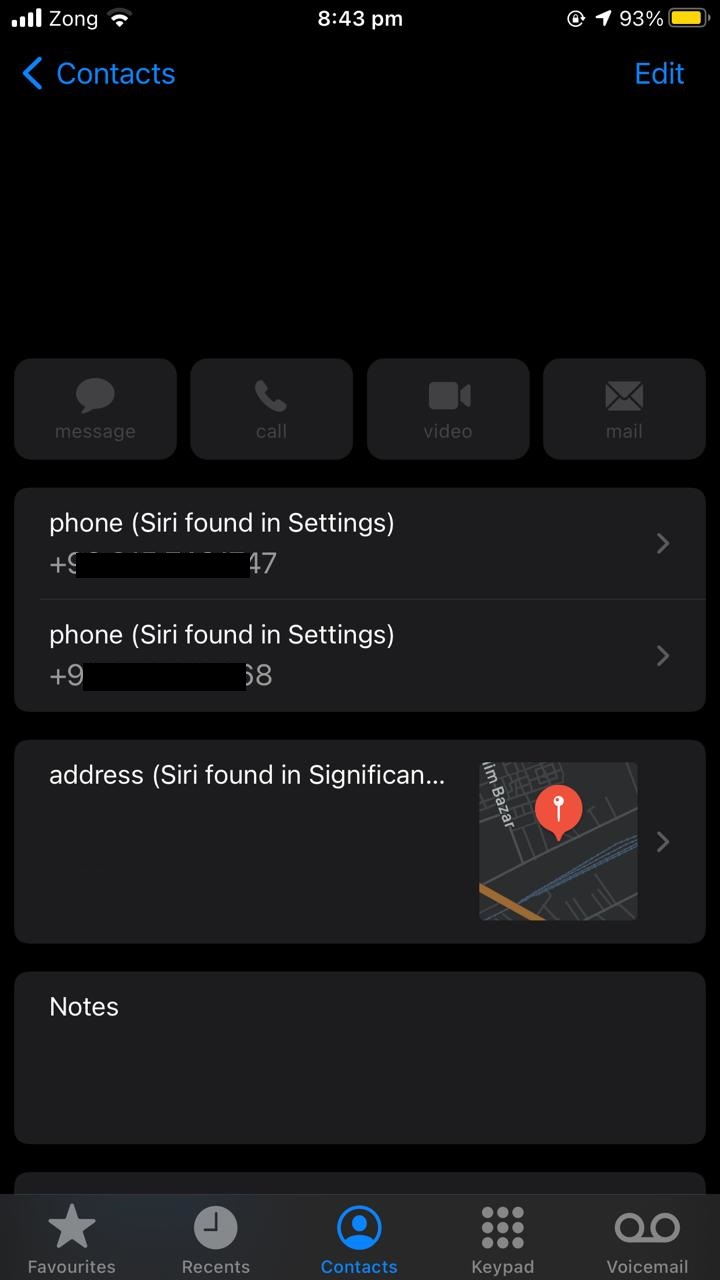Screenshot Description:

The screenshot is taken from a smartphone interface, showcasing the Contacts section of a phone application. The time is prominently displayed as "8:43 PM" at the top center of the image, with a battery life indicator showing 93% located in the upper right corner. The entire background of the screenshot is black, providing a stark contrast to the foreground elements.

In the upper left corner, there's a blue left-pointing arrow accompanied by the word "Contacts," also in blue. On the opposite side, in the upper right corner, the word "Edit" appears in blue. Below these elements is a blank space, followed by four rounded-corner rectangles arranged horizontally. Each rectangle bears a label and an icon: "Message" with a speech bubble icon, "Call" with a phone icon, "Video" with a video camera icon, and "Mail" with an envelope icon.

Below these options, white text reads "Phone Siri found in settings" with a phone number that has been blacked out for privacy. This pattern repeats with another blacked-out phone number under the same heading. Further down, the text "Address Siri found in significant" appears, trailing off into a partially visible context. This section is accompanied by a square map featuring a red pin, indicating a location.

At the bottom of the screenshot, more white text reads "Notes," followed by a menu bar at the very bottom. This bar displays five options: "Favorites," "Recents," "Contacts" (highlighted in blue), "Keypad," and "Voicemail," each with their respective icons above the labels.